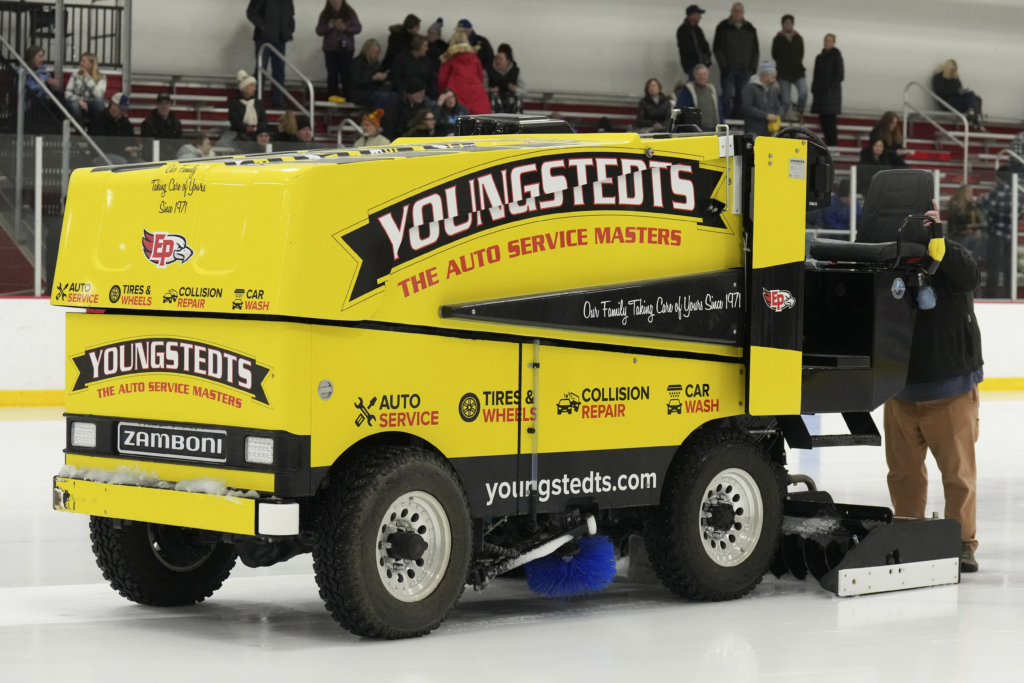In this image, we are at an ice skating rink where a bright yellow Zamboni, a boxy, rectangular-shaped machine used to clean and even out the ice, is prominently featured. The Zamboni has a distinct black trim and a banner on its side with white lettering that reads "Youngsteads, The Auto Service Masters." Below this, several services provided by Youngsteads are listed, including Auto Service, Tires and Wheels, Collision Repair, and Car Wash, likely serving as advertisements for the viewers in the stands. A man, dressed in cargo pants and a bluish shirt, is standing partially obscured behind the Zamboni, possibly making adjustments. The rink itself is pristine, with shiny white ice, and there are stands filling up with people in the background, set against white walls. The Zamboni's operative features, such as the driver's seat, the planer, and the brushes, are visible, emphasizing its function on the ice.